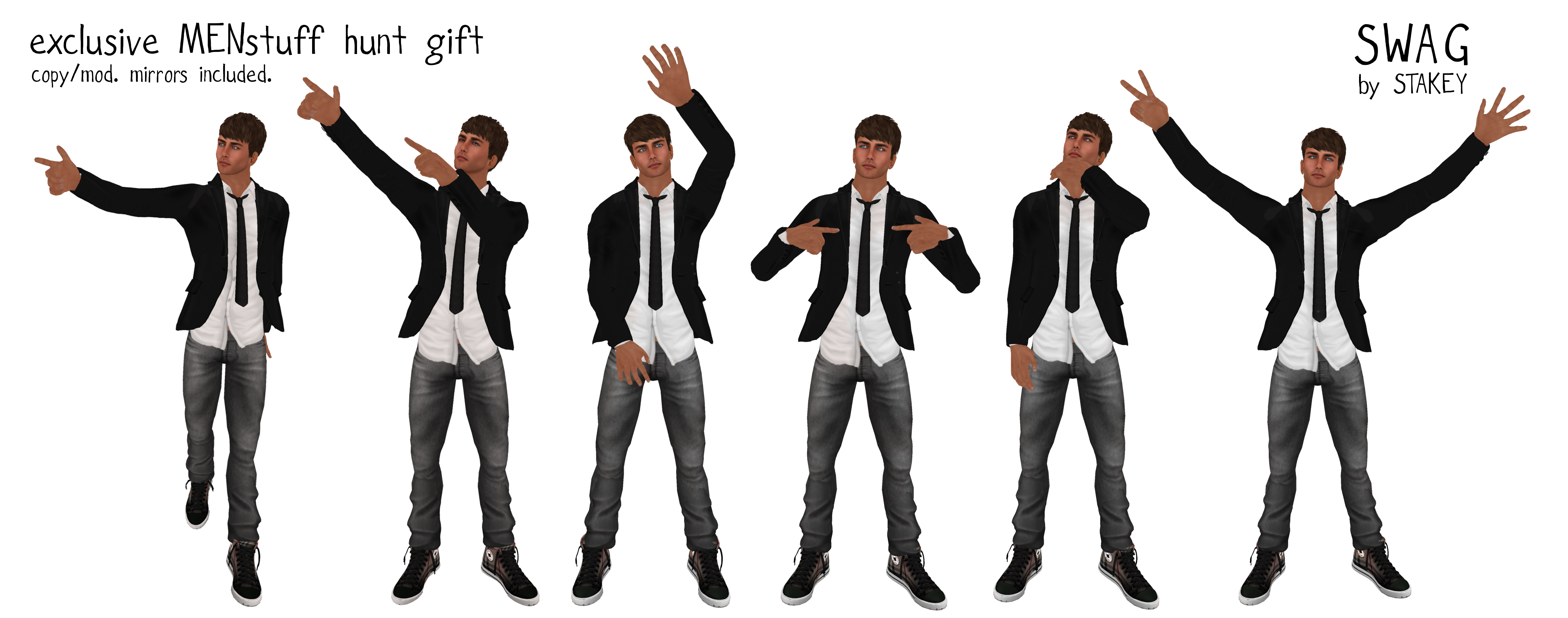The image depicts six 3D rendered men, who appear identical, against a white background. Each man is dressed in a black suit jacket, white shirt, black tie, gray pants, and black and white sneakers. The men are positioned horizontally across the image, each striking a unique pose. 

Starting from the left, the first man points to the right with his right arm, thumb and index finger extended. The second man points both hands upward, towards the sky. The third man raises his left hand with his palm facing forward while his right hand is down. The fourth man points at himself with his index fingers, drawing attention to his tie. The fifth man has his left hand on his chin, striking a thinking pose, while his right hand rests at his side. The sixth and final man on the far right extends both hands above his head, making a peace sign with his right hand and spreading all five fingers on his left hand.

In the upper left-hand corner, black text reads "EXCLUSIVE MEN'S STUFF HUNT GIFT" with "MEN" in all caps. Below this, it says "COPY / MOD, MIRRORS INCLUDED". In the upper right-hand corner, black text in all caps reads "SWAG BY STAKEY".